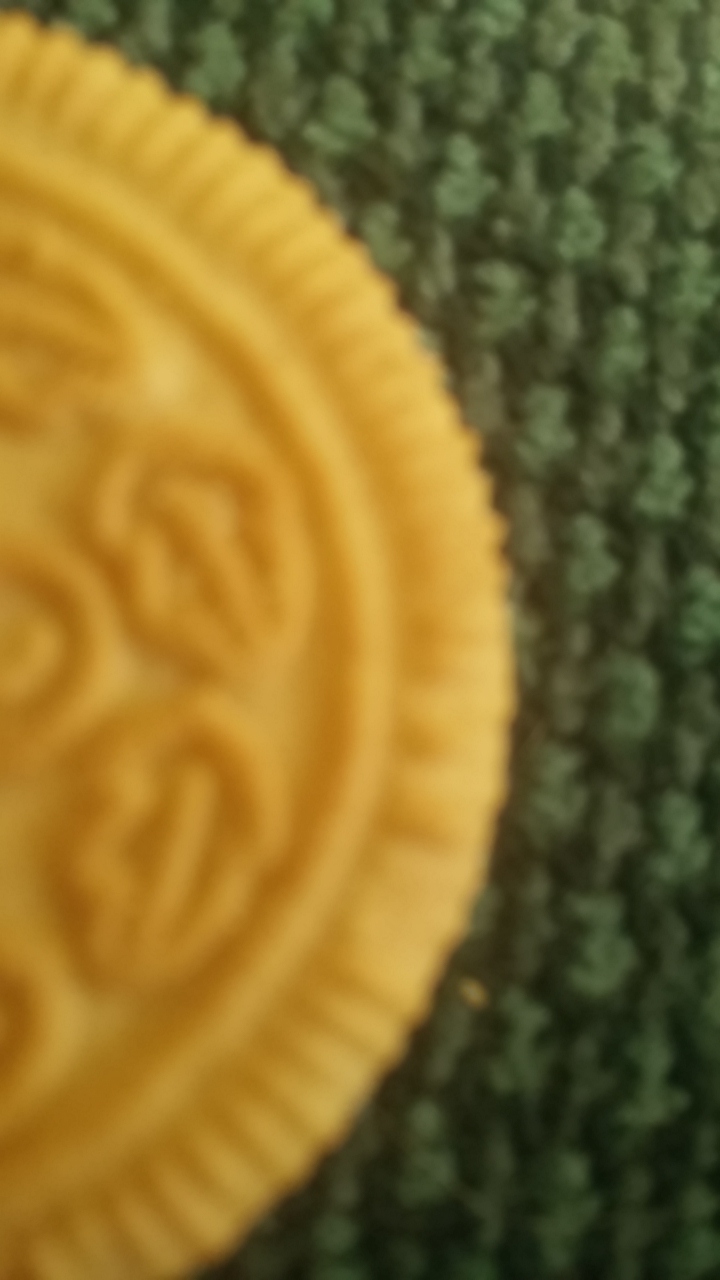The blurry image depicts a golden vanilla Oreo cookie with distinctive leaf imprints and ridges along its circular border, giving it a sun-like appearance. The cookie is prominently featured in the left half of the photo, though not fully in focus or within the frame. It rests on a green, textured knit item, possibly a blanket or rug, likely suggesting the photo was taken in a home environment, perhaps a living room.